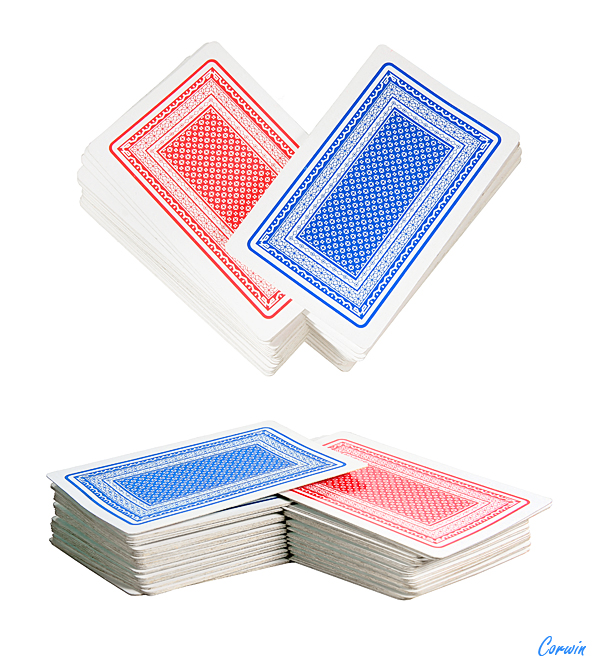A professionally taken product photograph features two stacks of playing cards meticulously arranged. The upper portion of the image displays a stack of red cards intersecting with a stack of blue cards, creating a visually appealing crisscross pattern. The cards are prominently highlighted, showcasing their vibrant colors and crisp edges. Additionally, discernible in the bottom corner of the image is a subtle watermark belonging to a company named Corwin, adding a touch of branding to the composition. Overall, the arrangement and quality of the photograph highlight the product's aesthetic appeal and craftsmanship.